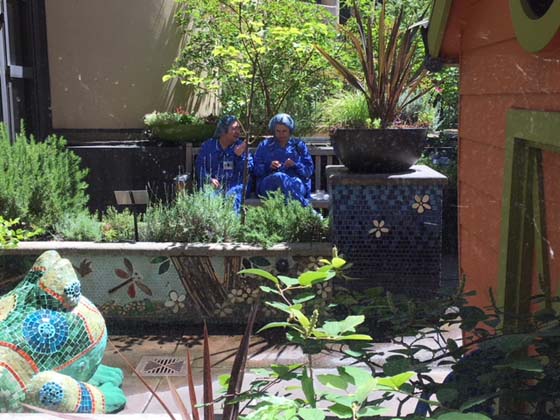This photograph captures a vibrant and detailed setting in what appears to be an urban garden or outdoor waiting area. Two people, dressed in blue jumpsuits and matching blue hair covers, sit side by side on a gray bench situated against a gray partition wall, likely taking a break from work or a medical procedure. The immediate foreground showcases a rich assortment of plant life, including green leaves and a brown spiky plant. To the left, a colorful ceramic tile design of a frog with pointy eyes and blue circles adds a whimsical element. The ground beneath is a brown cement slab. 

The scene extends to a planter wall in the background, adorned with a mosaic tile design depicting a dragonfly, a tree, and flowers. Adjacent to this, a striking blue ceramic tile post, embellished with white flower designs, supports a large black rounded vase with another brown pointed plant sprouting from it. The overall mood is bright and sunny, suggesting this tranquil and artfully decorated garden offers a peaceful respite for its visitors.